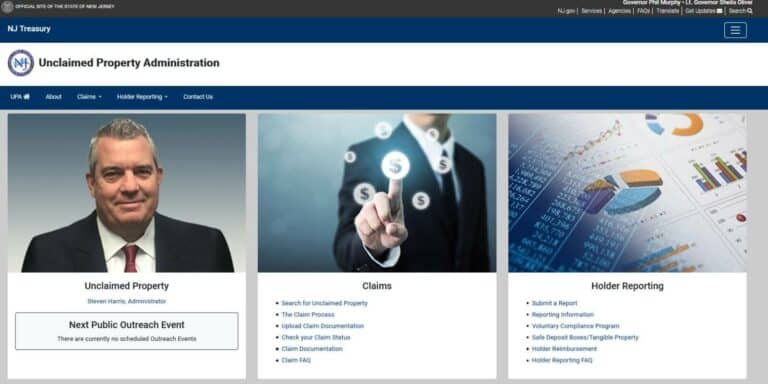This image, sourced from the NJ Treasury Unclaimed Property Administration website, prominently showcases various elements related to unclaimed property and public outreach. On the left, there is a smiling man, likely around 52 years old, with gray hair. His head and shoulders are visible, and he is dressed in a formal black suit paired with a red tie and a white collared shirt. Beneath this section, text reads "Unclaimed Property - Next Public Outreach Event."

On the right, another visual element features the lower face of a man, specifically his chin and neck, as he points towards a prominent dollar sign. Surrounding this central dollar sign are several other dollar signs, creating a focal point symbolizing financial claims. Adjacent to this image, the text "Holder Reporting" appears, alongside a button designed for submitting a report. The overall composition effectively communicates information regarding unclaimed property claims and reporting procedures.